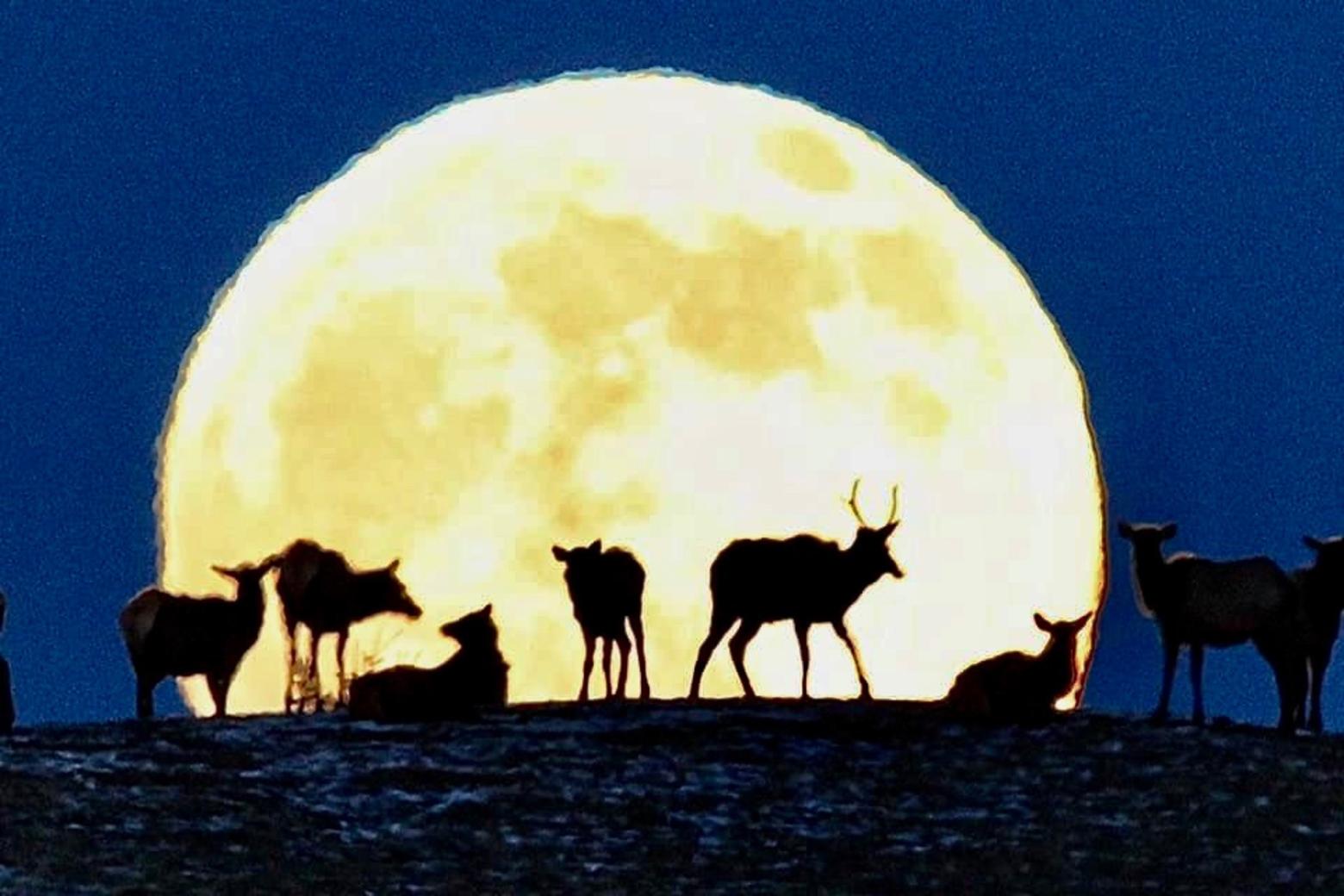The image appears to be a highly detailed painting, capturing a surreal and atmospheric night scene. Dominating the background is an enormous, glowing full moon that seems to consume almost 70% of the frame, its lower portion obscured by the horizon. The moon's luminescence casts the night sky in a rich, dark blue hue, speckled with lighter patches. The scene's palette consists primarily of blues, light tans, and yellows, creating a mood of serene stillness.

In the foreground, the ground appears rugged and slightly rocky, rendering it in dark, bluish-black tones with the occasional white splotch. Amidst this rugged terrain, silhouetted against the radiant moon, stand a group of eight deer. These deer are portrayed in various postures; some are standing while others are lying down. Their forms are primarily dark outlines, one of which features prominently large antlers, suggesting a stag. The detailed composition, notable for its contrasts and shadows, offers a mesmerizing interplay between the illuminated night sky and the silhouetted animals, evoking a scene of tranquil wilderness at night.